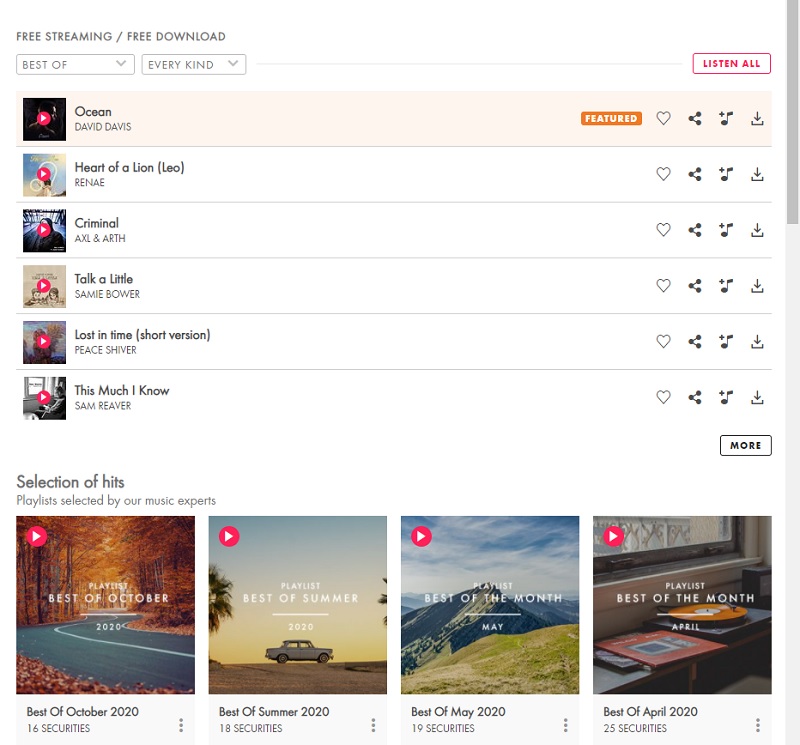This image showcases an intuitive and feature-rich interface for a free music streaming and download website. The interface prominently displays various filters and options to enhance the user experience. The primary section features a curated list of tracks, beginning with "Oceans" by David Davis, marked as a featured song. 

To the left of each track, a play button allows users to listen to the music, with an option of audio or possibly video playback. Adjacent to each track title, there are icons for liking (heart), sharing, adding to a playlist (music with a plus), and downloading. 

Highlighted tracks include "Heart of a Lion" by Renée, "Excellent Earth" by Criminal, "Talk a Little" by Sammy Bauer, "Lost in Time" (short version) by Peace Shiver, and "This Much I Know" by Sam Reaver. 

At the bottom of the page, a selection of expertly curated playlists is presented, featuring collections such as "Best of October," "Summer Hits," "Best of the Month," and "Best of April." 

Additional navigation options include filtering music by genre or preference, with a "Best of the Best Music" category accessible via the filter panel. On the far right, users can access the “Listen All” button, highlighted in red, allowing for continuous play of selected tracks or playlists. 

The layout is designed to be user-friendly, providing easy access to music discovery and playback, catering to enthusiasts looking for both specific tracks and expertly curated playlists.